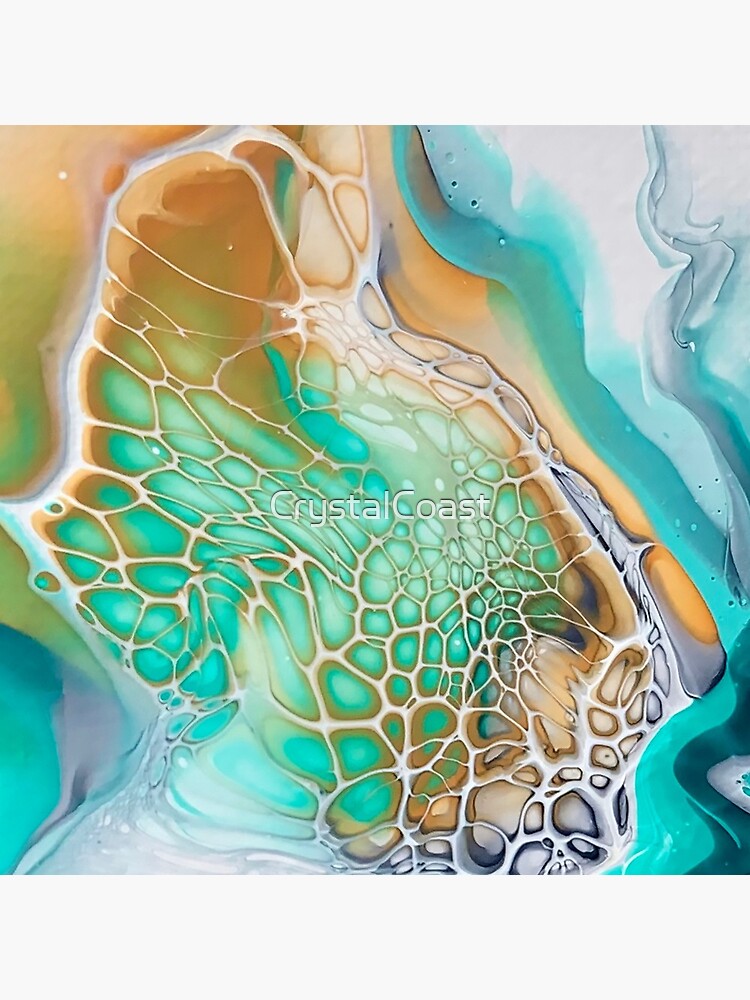This is an abstract cartoon diagram that blends oil and fluid, featuring an intricate and organic design reminiscent of cell divisions often seen in bones and plant cells. The image displays a beige, web-like structure overlaying a mix of turquoise blue, orange, and white fluids, creating a coastal appearance. This fluid, swirling pattern evokes the look of poured acrylic paint, resulting in a random, splattered effect. The upper right section contains whitish and teal hues with a teal squiggly line running diagonally, while the upper left showcases a yellow-gold color. The middle and bottom sections predominantly feature teal and white, forming an intricate web-like pattern. The entire composition, characterized by wavy, curvy lines, and trypophobia-inducing holes, centers around white text reading "Crystal Coast" with a black drop shadow, giving a clear focal point within this square image.